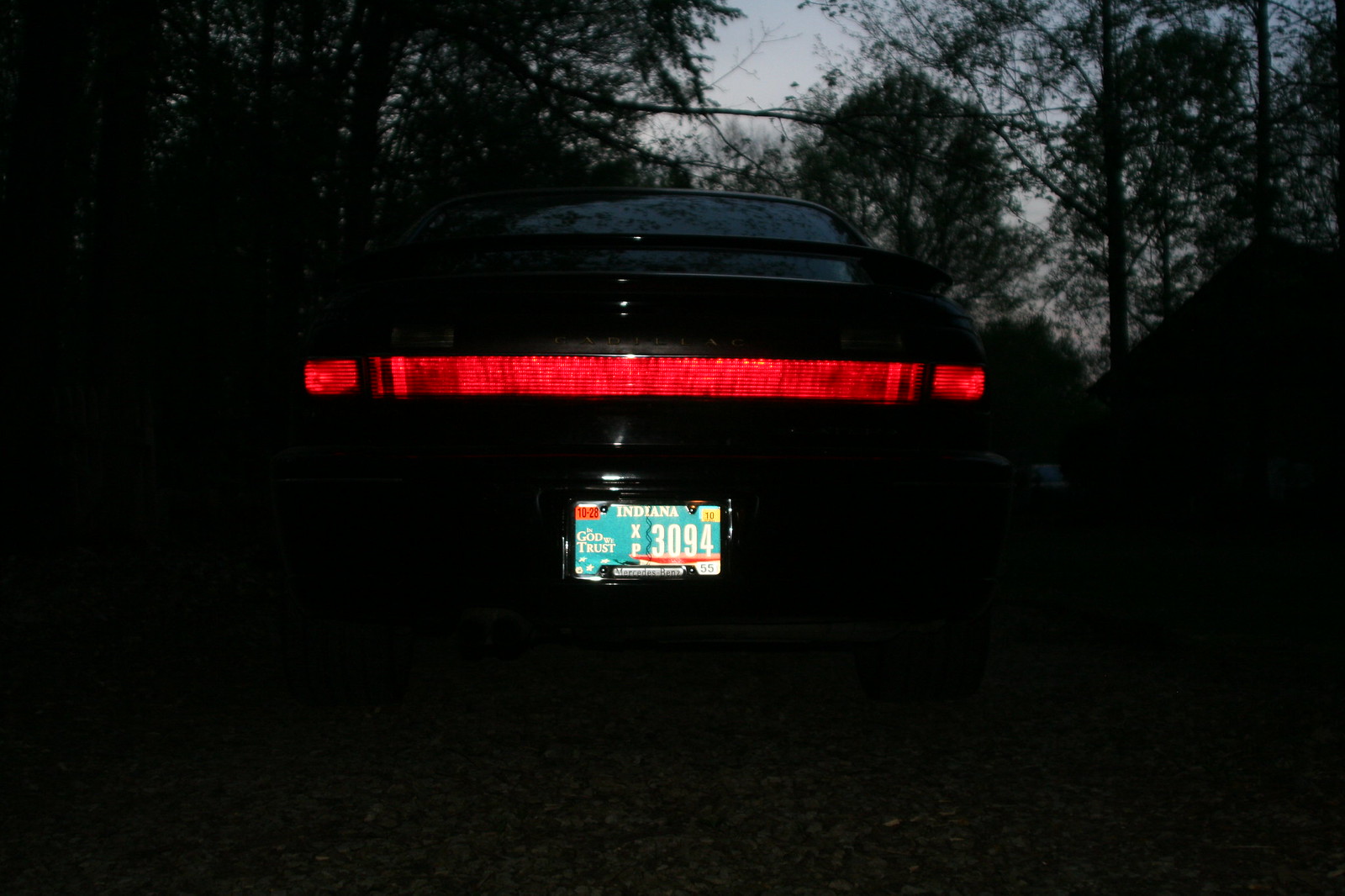The image captured at night depicts a black car parked in a densely wooded area. Its windows are tinted black, adding to the vehicle's mysterious appearance. The most distinctive feature is the uninterrupted red brake light stretching entirely across the back. The car's license plate, illuminated, stands out with a teal color and white lettering, revealing partial text indicating it's from Indiana, with discernible elements including "XP" at the top, “3094” in the middle, and additional details like a yellow sticker in the upper right corner and the phrases "In God We Trust" and "Mercedes-Benz" in a white rectangle. Surrounding the car are numerous trees casting dark silhouettes against a dusky sky that isn’t quite pitch black, creating a shadowy, secluded atmosphere. The car appears to be parked on a surface resembling small rocks or pebbles, further obscured by the dim light.